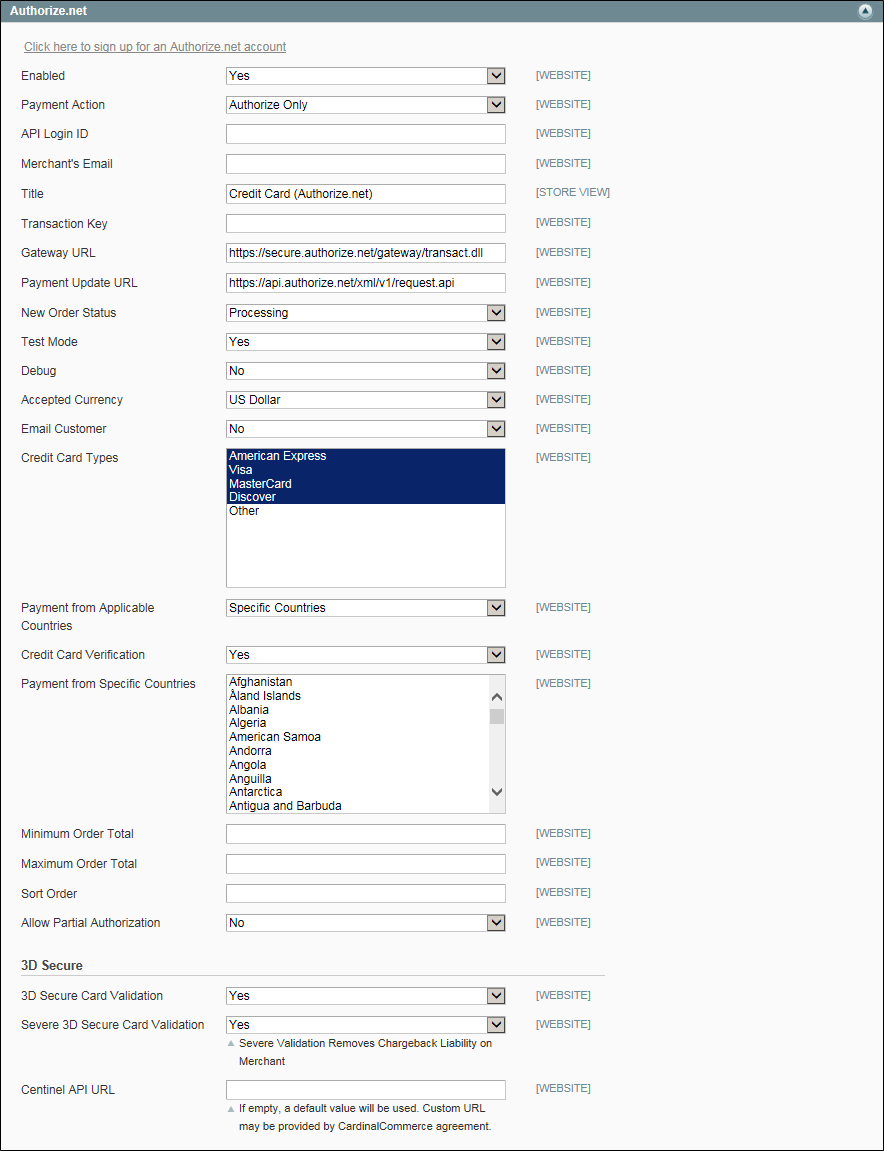The image depicts an authorization screen filled with a long list of drop-down menus and various settings. At the top left, the text "Enabled" is displayed in black, and the corresponding drop-down menu is set to "Yes". Moving to the right, there's another drop-down field labeled "Website", which is hyperlinked.

To the options section, the leftmost field says "Enabled" again. Directly below that, there's a label saying "Payment Action" with the setting "Authorize Only" to the right. The next drop-down box down is labeled "API Login ID", but it is empty. Below this, there's a field labeled "Merchant's Email", which is also unfilled.

Continuing rightwards, the next field down is labeled "Title" and is showing "Credit Card". Below this, there's a field labeled "Gateway URL" set to a secure authorized URL. Beneath that, "Payment Update URL" appears with another URL filled in next to it.

The drop-down menu under "Processing" is set to "No". Similarly, the field labeled "Test" also has its drop-down menu set to "No". The "Debug" field has a drop-down menu set to "No" as well. 

Further down, the field labeled "Accepted Currency" has a drop-down menu displaying "US Dollar". Below this, "Email Customer" has a drop-down menu set to "No". Finally, "Credit Card Types" lists multiple options such as American Express, Visa, MasterCard, and Discover - all selected.

The background of the screen is a light gray, with selected texts and options appearing in dark blue. There are additional settings and options further down the screen.